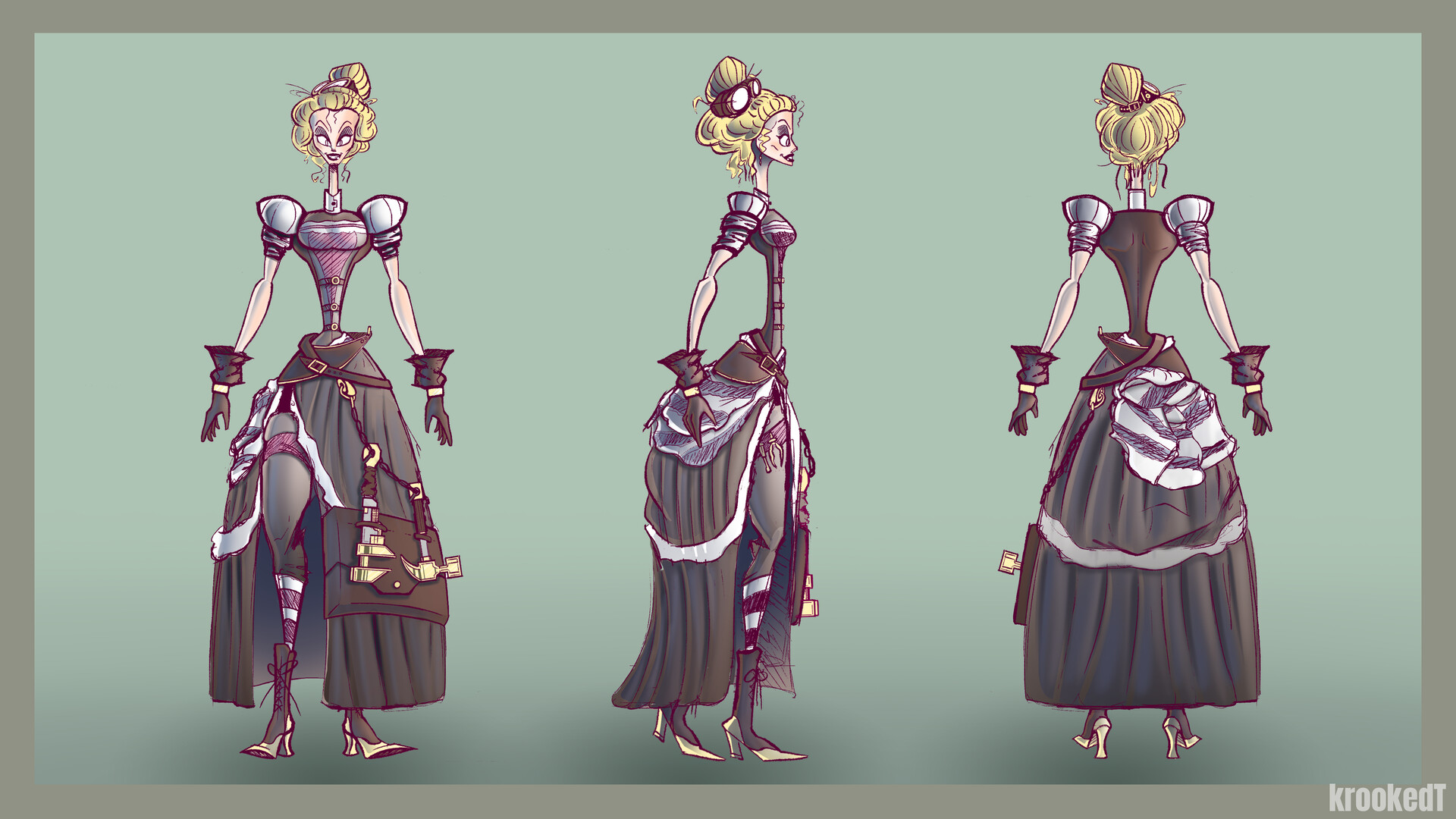This artwork features a trio of stylized female figures depicted in three different positions within a gray frame against a light olive green background. Each figure, with elongated necks and abdomens, exudes a peculiar yet striking Victorian-inspired aesthetic. The central figure is dressed in a dramatic outfit with an ankle-length skirt that features a slit extending up to the waist, accentuated by yellow high heels and elbow-length dark gloves. She sports a tiny waist, puff sleeves, and a magenta bodice adorned with intricate detailing. Her face has sharp features, and she wears a high blonde hairdo, complete with a magenta hairband and goggles or binoculars perched atop her head. The figures are depicted with unnaturally long, insect-like proportions, and their waists are extraordinarily narrow, resembling that of a bee, adding to their surreal appearance. The artwork captures the front, side, and back views of the figure, with the back view emphasizing the dress's bustling detail. The perplexing nature of the image is further underscored by the unsettling proportions and the inscrutable expression on each figure’s face, lending a futuristic, almost mechanical vibe. The piece is signed “EDT” in the bottom right corner, marking the artist's unique, otherworldly vision.